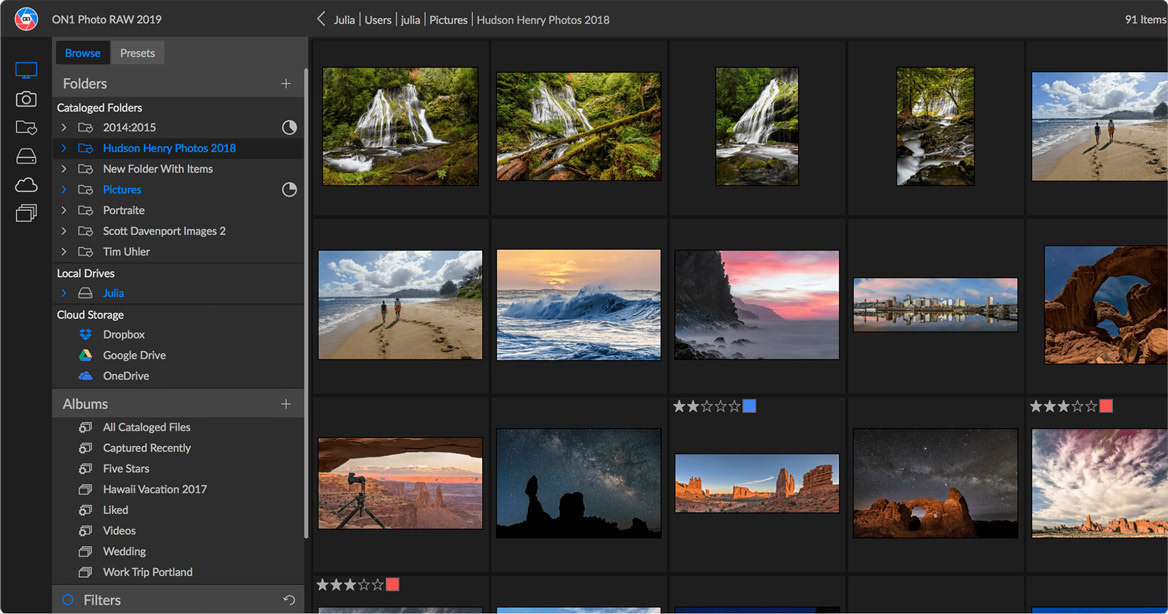This is a detailed screenshot in night mode, featuring a black background with light gray highlights from the ON1 Photo RAW 2019 application. The prominent ON1 logo is visible at the top, showcasing its distinctive blue and red colors. The path displayed at the top reads: "Julia > Users > Julia > Pictures > Hudson > Henry > Photos > 2018". On the left side, there's a menu with a dropdown selection of various photo albums and cloud storage options. The currently selected album is "2014 Hudson Henry Photos". Other entries in the menu include "New Folder with Items", "Pictures", "Portraits", "Scott Davenport", "Images 2", and "Tim Uth-Uller".

To the right, the main panel displays an array of stunning nature photographs. The top images depict a serene waterfall set amidst a lush forest, followed by scenes of a beach with people walking along the shore, dynamic waves crashing, and a breathtaking sunset on a rugged coastline. Further down, there is an urban city skyline, a typical Arizona desert landscape with striking natural rock formations, and an awe-inspiring starry night sky captured in the heart of the desert. The text in the menus helps to effortlessly navigate through the various options and albums. This comprehensive layout allows the user to enjoy and manage their photographic collections with ease and elegance.